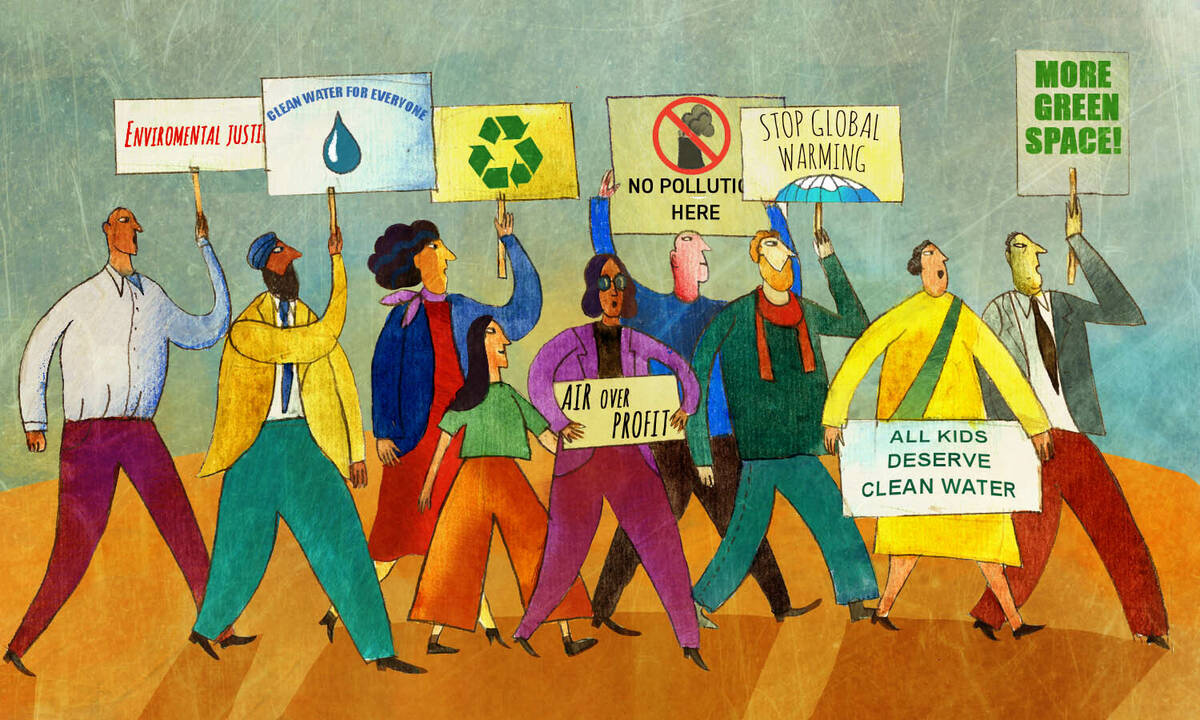The image portrays a vibrant, stylistic cartoon painting or drawing of a diverse group of protesters advocating for environmental causes. The exaggerated figures, featuring small heads and large bodies and limbs, include approximately 10 to 13 individuals of varying ethnic backgrounds, including a white man, an Indian Sikh man, black and white women, among others. They are dressed in colorful, office-like attire, often in suits, skirts, and ties. 

The protesters are marching forward, each holding signs attached to yellow sticks. The signs display messages such as "Environmental Justice," "Clean Water for Everyone," "Stop Global Warming," "No Pollution Here" with a smokestack crossed out, "Air Over Profit," "All Kids Deserve Clean Water," "More Green Space," and a recycling symbol. 

The scene is set against a blue background with a brownish-orange ground, and the characters’ clothing features a range of primary and basic colors, including yellows, greens, reds, purples, and blues. Despite the flat, non-dimensional appearance, the image is rich in detail and vibrant in its depiction of a passionate environmental protest.